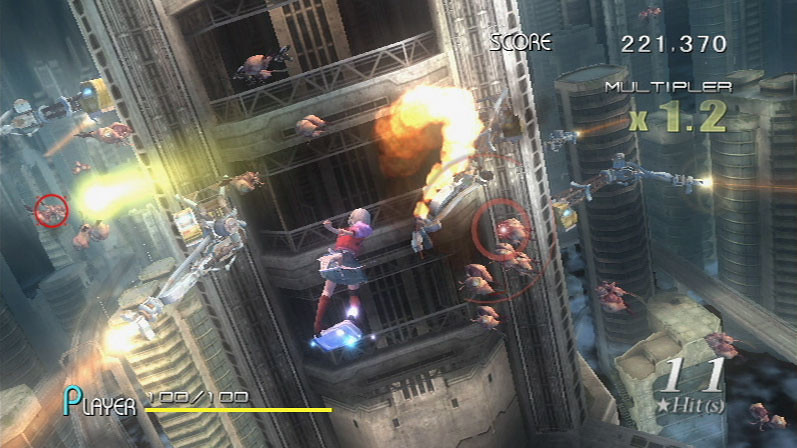In this vivid screenshot from a futuristic video game, we are given an aerial view of a sprawling metropolis. Tall skyscrapers dominate the scene, constructed predominantly from concrete and adorned with numerous windows. The city's architectural marvels create a striking juxtaposition against the sky, which is filled with a multitude of characters flying in various directions. 

At the heart of the image, one building appears to be on fire, with bright flames adding to the chaotic atmosphere. The game's score is prominently displayed, reading 221,370, while the player's health is at a perfect 100 out of 100. Alongside this, a "one hit" notification suggests recent successful actions.

The color palette is a dynamic mix, featuring vibrant blues, reds, and oranges, which particularly highlight the blazing fire and flying characters. These colors stand out against the prevalent shades of gray and black that define the city's structures. Among the myriad of flying figures, some characters are marked with red targets, indicating they are likely adversaries.

This detailed snapshot captures the essence of the game's high-energy environment and the player's active engagement within this futuristic urban battleground.